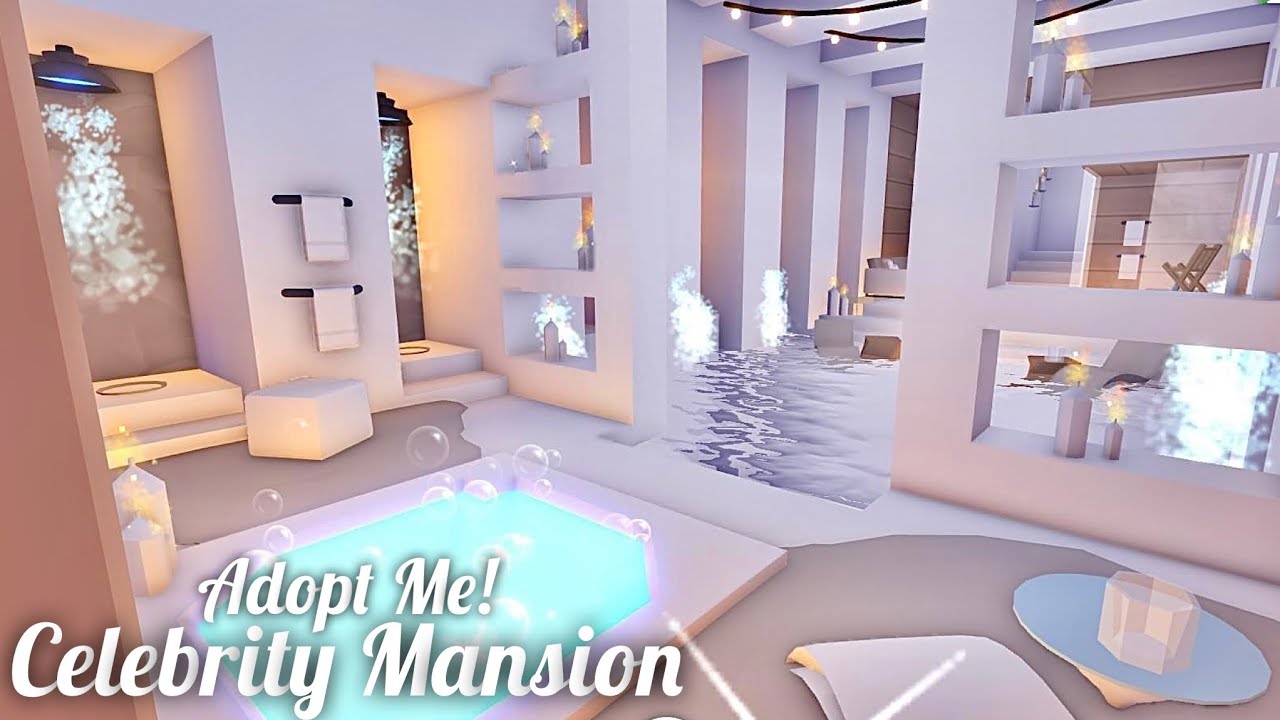The image showcases a luxurious and modern spa room, likely a screenshot from a video game or mobile app aimed at younger audiences, entitled "Adopt Me! Celebrity Mansion," as indicated by the white text in the bottom left-hand corner. The room is adorned with a spacious spa pool bubbling energetically in the center. In the background, a large rain forest shower head releases a steady stream of water into the shower area. The water from the pool seamlessly flows into the main area, creating a lavish, step-down pool ambiance. The room is further embellished with top-mounted lights and rectangular holes cut out of the walls, giving an open, connected feel across various spaces. Candles are lit around the pool to enhance the serene atmosphere, with a gentle smoke rising, adding to the overall relaxing vibe. The scene is completely devoid of people, emphasizing the tranquility and exclusivity of this beautifully crafted virtual space.